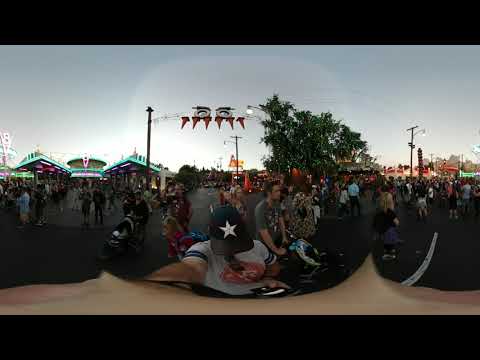The image captures an outdoor event at dusk, where the sky is darkening but still illuminated near the horizon. The photo, taken with a 360-degree fisheye lens, centers on the photographer, whose face is obscured by a black baseball cap with a white star. He is wearing a white t-shirt with blue stripes on the sleeves. His arm dominates the foreground due to the lens effect. Behind him, a vibrant scene comes to life with numerous people milling about on a wide street or pedestrian walkway, which could be a carnival or similar gathering. The atmosphere suggests warm weather, with attendees clad in shorts and short sleeves, and some pushing prams. Structures adorned with neon lights, featuring blue and red hues, illuminate the backdrop, alongside a building with neon-lit edges and a cylindrical centerpiece. To the right, tall trees frame the scene, almost reaching a banner strung between two poles, possibly marking the event's entrance. The photo's panoramic nature provides a broad view, capturing the lively crowd and the brightly lit surroundings.